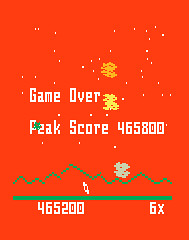This detailed vertical screenshot from a video game features a vivid red-orange background with a plethora of white dots scattered across the top, resembling a starry night. Dominating the image is the text in white letters, "Game Over," followed by "Peak Score: 465,800" on the next row. Below this, a distinct green, mountainous horizon stretches across the screen, with a solid green line right above it. Below this green line is an additional score of 465,200. On the right-hand side of the screen, "6X" in white text is visible. Adding to the visual complexity, there are three small blotchy sections in various colors—gold, yellow, and light blue—creating a layered color effect. Near the bottom, several shorter green lines extend upwards, enhancing the imagery of a mountainous terrain.